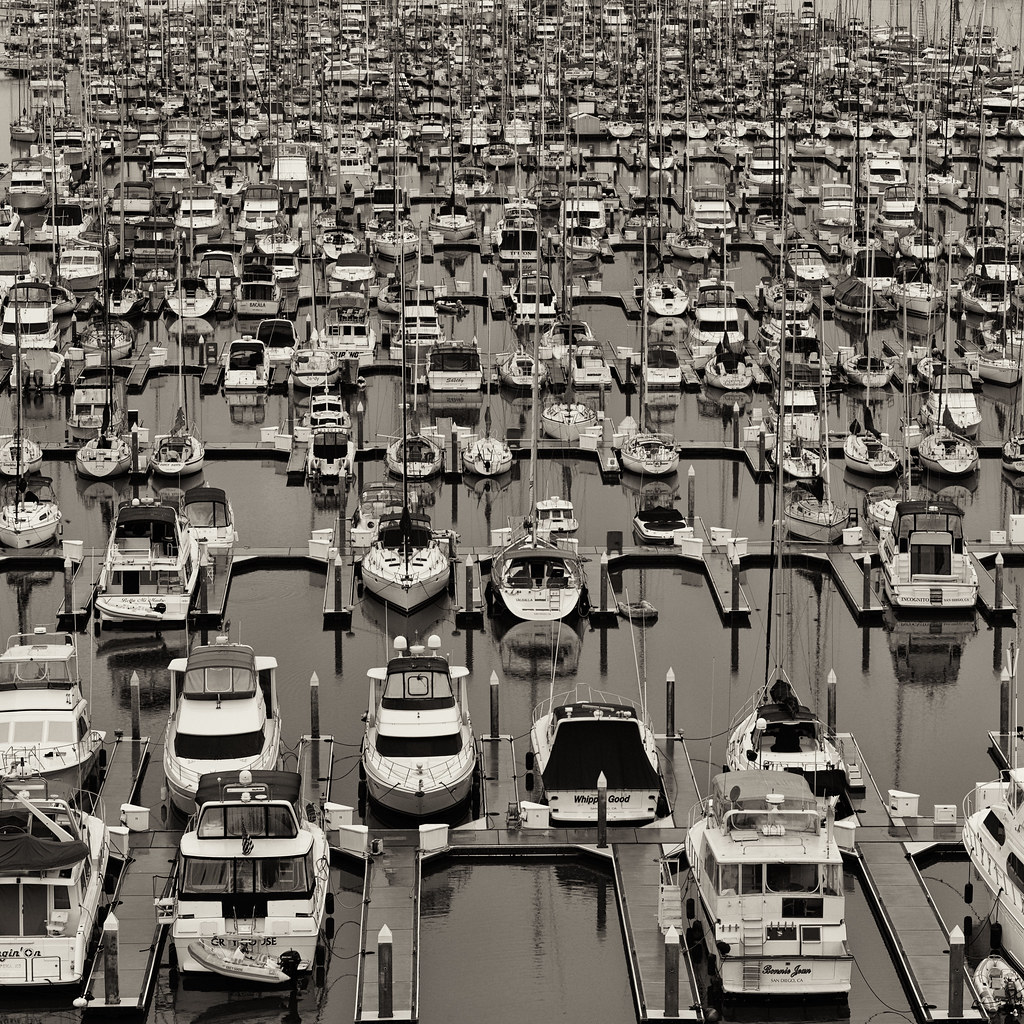This detailed black-and-white aerial photograph, taken from approximately 80 to 100 feet above, captures a bustling marina densely packed with boats and docks, spanning the entire width of the image. The marina is teeming with various types of boats, predominantly motorized personal pleasure boats, alongside a smaller number of sailboats identifiable by their tall masts. The boats vary in size and design, with some featuring two levels and covered cabins, while others are open. The foreground displays a mix of docks and a few boats, but as the image extends towards the background, the scene becomes increasingly crowded with boats, virtually obscuring the water beneath. Each dock is lined with many boat slips, heavily populated with boats—possibly three or four hundred in total. Despite the grayscale nature of the photograph, the intricate details of the marina infrastructure, such as cement posts for floating docks and walkways for access, are clearly visible, emphasizing the sheer density and variety of boats present in this lively nautical setting.